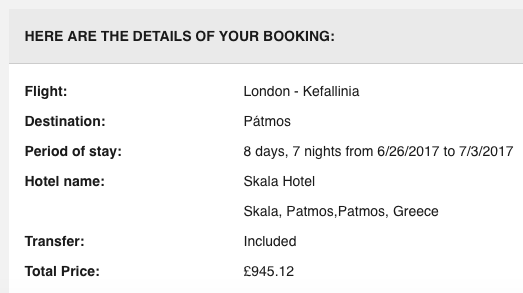The photograph captures a screenshot primarily featuring a monochromatic color scheme dominated by white, gray, and black tones. At the top, a gray banner prominently displays black, all-caps text stating, "HERE ARE THE DETAILS OF YOUR BOOKING." Below this banner, the background shifts to white with black text presenting the booking information. It details a flight originating from London to Keyfilenia, with a destination of Padmos. The stay period is clearly outlined as 8 days and 7 nights, spanning from June 26, 2017, to July 3, 2017. The hotel information is also provided, specifying the accommodation as Scala Hotel, located in Padmos, Greece. Additionally, it indicates that the transfer is included. The total cost for this booking is €945.12.